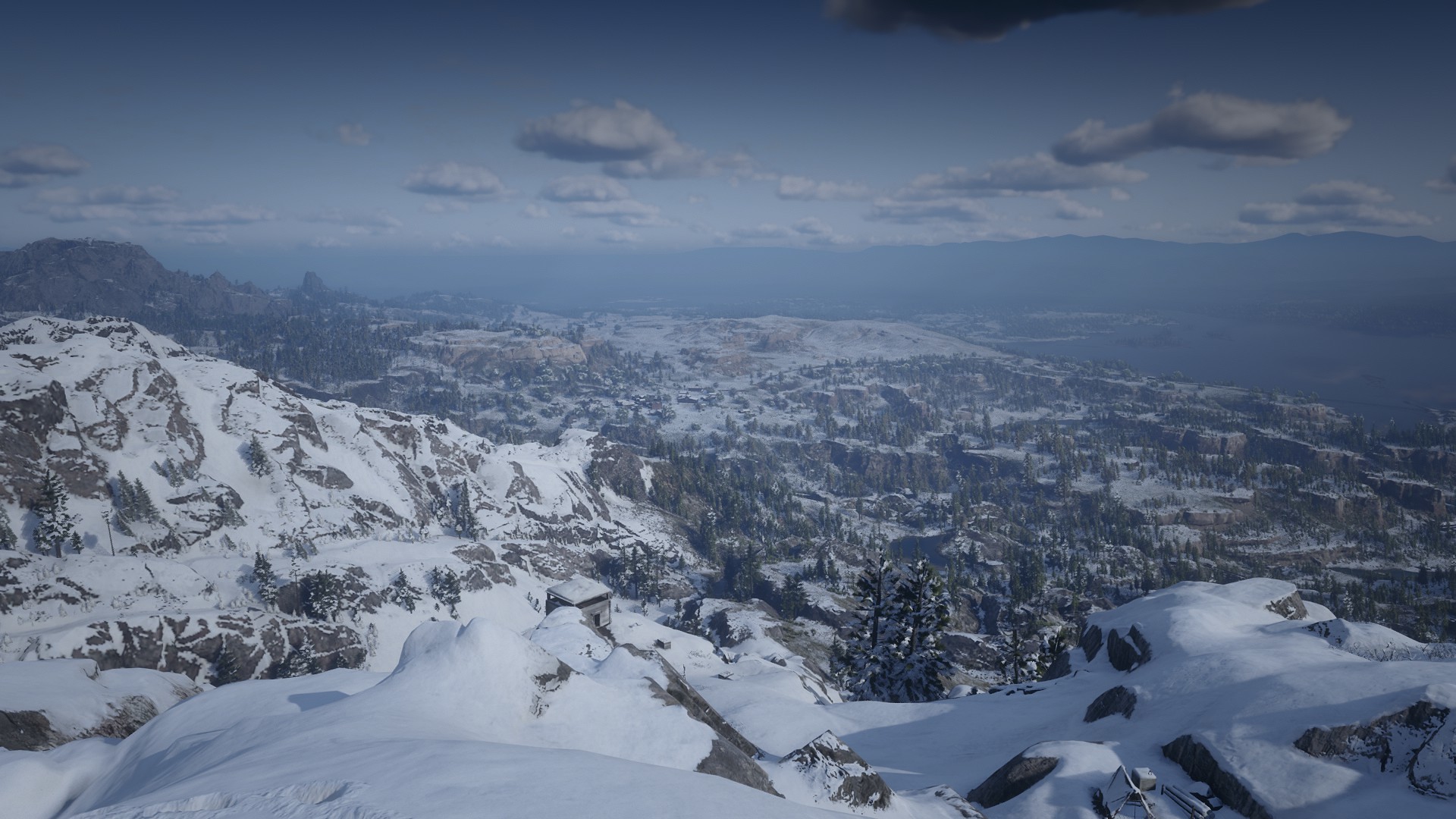A breathtaking photograph captured from a lofty peak in a snowy mountainous region, possibly in Colorado or another snow-laden locale. The landscape is engulfed in a pristine blanket of snow, interspersed with rugged hills and dense clusters of evergreen trees and rocky outcrops. In the foreground, the snow-draped terrain dominates, while scattered buildings peep through the white expanse, hinting at human habitation. Far in the distance, additional towering mountains rise against the horizon, their majestic presence softened by the haze. A glistening body of water can also be discerned, adding a serene contrast to the wintry scene. The overall vista is one of serene, untouched natural beauty, encapsulating the tranquil and awe-inspiring essence of a high-altitude winter wonderland.